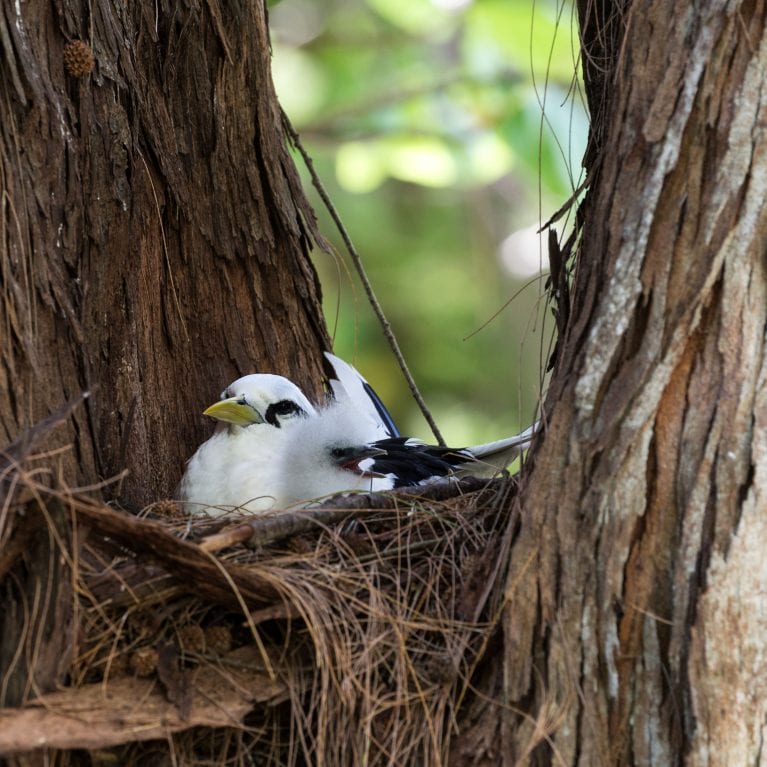This close-up image captures a striking scene of a predominantly white bird with a yellow beak and black markings, nestled comfortably between two tree trunks. The bird's detailed features, including its black-tipped wings and black markings around its eyes, are clearly visible. It sits serenely on its nest, which is constructed from twigs and dead grass, meticulously placed at the V-shaped split between the tree trunks. The bark of the tree is sharply detailed, revealing a string-like texture where the tree appears to have split. In the blurred background, shades of green and brown hint at a woodland setting, with some foliage and perhaps pine cones, suggesting the trees might be pine. The bird is slightly off-center, gazing towards the left of the image, creating a peaceful yet compelling composition.